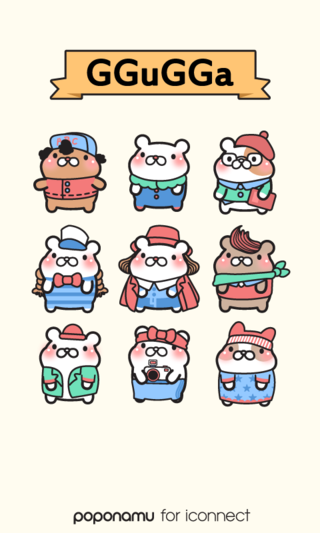The illustrated image, rendered digitally, showcases a portrait-oriented scene with a cream background. At the top of the image, there is a golden-yellow ribbon-style banner featuring the text "GGUGGA," with the G's in uppercase and the u and a in lowercase. At the bottom, there is another piece of text that reads "Poponamu for iConnect" in lowercase letters.

The central focus of the image is a grid layout of nine anthropomorphized characters, arranged in three rows and three columns. These characters resemble bears or possibly hamsters and are depicted in various skin tones and attire. The top-left character is distinct with darker brown skin, a blue hat worn backward, and an orange shirt. Other characters include a bear with white skin, red cheeks, and green overalls, and another with a red beret, glasses, and a green sweater holding a bag. Additional characters wear items such as a bow, top hat, cape, and camera, showcasing a wide array of personalities and styles. The detailed clothing and accessories suggest a playful and diverse theme, reflective of the names and references like "GGUGGA" and "Poponamu for iConnect."